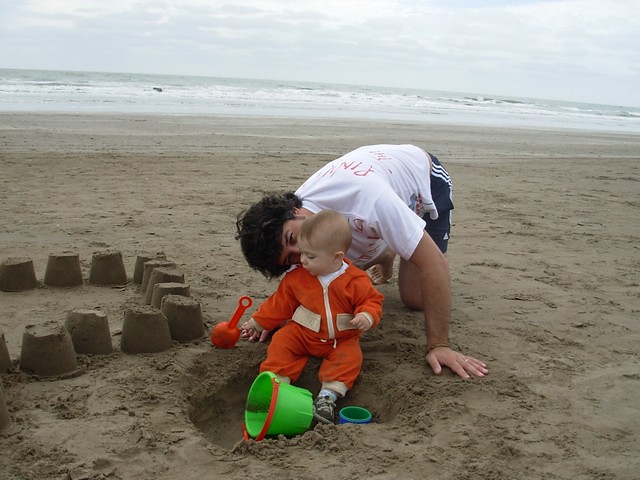The photograph captures a tender moment between a man and his very young child, likely under two years old, on a beach during the daytime. The background features a cloudy sky with a faint sliver of blue at the top, juxtaposed against a greenish ocean. The earthy brown sand contrasts with the not-so-vivid sky, setting a serene atmosphere.

In the foreground, the man is kneeling down, donned in a white t-shirt and blue pants or possibly blue and white striped shorts, with dark hair. He appears to be kissing the child, who is wearing an orange onesie. The child, with sparse hair, indicative of a young age, is playing with the sand, feeling it between his fingers. In front of the child is a little green plastic bucket and a tiny shovel, illustrating their sandcastle construction effort, characterized by rows of small, conical sand pieces forming a square castle circumference.

Besides the child is a bright orange toy, perhaps a spatula or spoon, and the boy is sitting near a small hole they've dug. The composition of the photo, with the affectionate interaction and the simple, playful beach setting, paints a heartwarming scene of familial bonding.